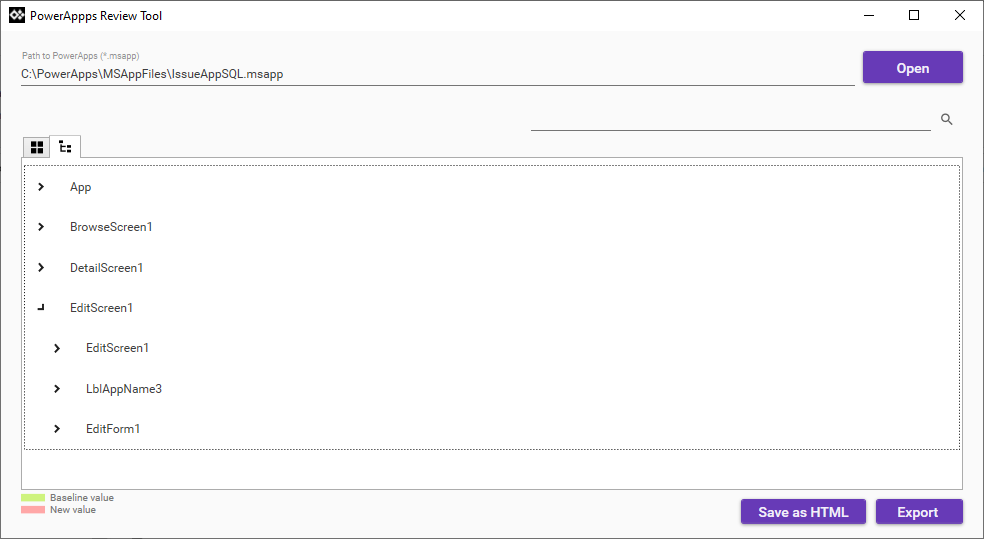This is a detailed caption for an image showcasing a Power Apps review tool interface:

---

The image displays a user interface of the Power Apps Review Tool set against a white background. At the top, a white navigation bar features a logo on the left portion which has a black background depicting two white symbols: a circle and a cross. Adjacent to the logo, the text "Power Apps Review Tool" appears in black letters. Beside this text are three icons for minimizing, maximizing, and closing the application respectively.

Below this bar, there's a label reading "Path to Power Apps" followed by a specific address that users can use on their computer to locate the Power Apps Review Tool. To the right of this is a purple button with white text that says "Open."

Beneath this section on the right side resides a search bar. Following this, there's a series of drop-down menus starting with "App," followed by "Browse Screen 1," "Detail Screen 1," and "Edit Screen 1." The "Edit Screen 1" menu is expanded, showing further options which include "Edit Screen 1 LL," "Bl App Name 3," and "Edit Form 1."

In the bottom left corner of the interface, a green bar labeled "Baseline Value" and a pink bar labeled "New Value" are visible. The bottom right corner contains options to "Save as HTML" or "Export."

---